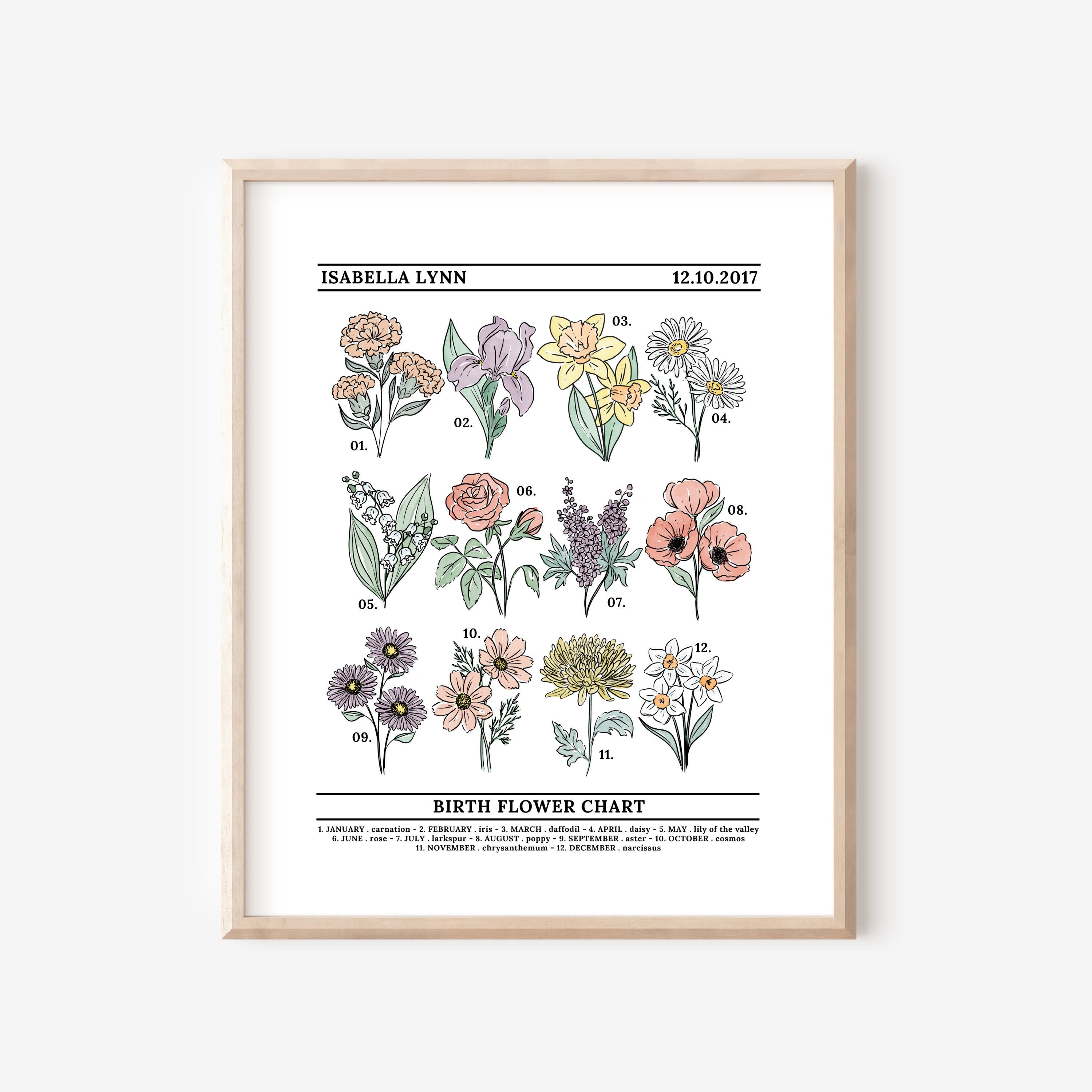The photograph showcases a framed poster titled "Birth Flower Chart," prominently placed on a wide white wall. The light brown wooden frame encloses a white background on which 12 colorfully illustrated flowers are displayed in three rows of four. Each flower, unique in its variety, represents a different month of the year and features soft pastel shades of pink, purple, yellow, white, and orange. Above the floral illustrations, in simple black print, the name "Isabella Lynn" is flanked by the date "12-10-2017" (October 12th, 2017). Each flower is labeled with numbers from 1 to 12, correlating with each month, and the poster's lower section includes the title "Birth Flower Chart" in black text along with a legend detailing each month's respective flower.